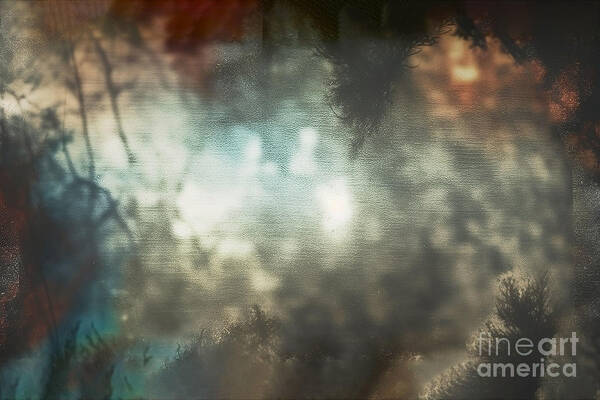This image appears to be a blurry, dreamy digital artwork or a photorealistic painting. The main focus is a forest scene, abstractly rendered to evoke a sense of ethereal reflection, as if viewed on the surface of water. Visible in the image are various natural elements such as pine needles, branches, and leaves, some of which are reflected in the hazy center, creating a diffuse, glistening effect reminiscent of sunlight filtering through a forest canopy. The colors predominantly comprise muted greens and browns, with bursts of rust orange, deep blue, and brighter oranges and reds toward the corners, suggesting the play of golden sunlight and shadow. A watermark reading "Fine Art America" in white text, with "Fine Art" in thinner print above a slightly thicker "America," is situated in the bottom right corner. Aspects like the triangular branch form or the pine needles on the edges add to the intricate texture of this evocative scene.